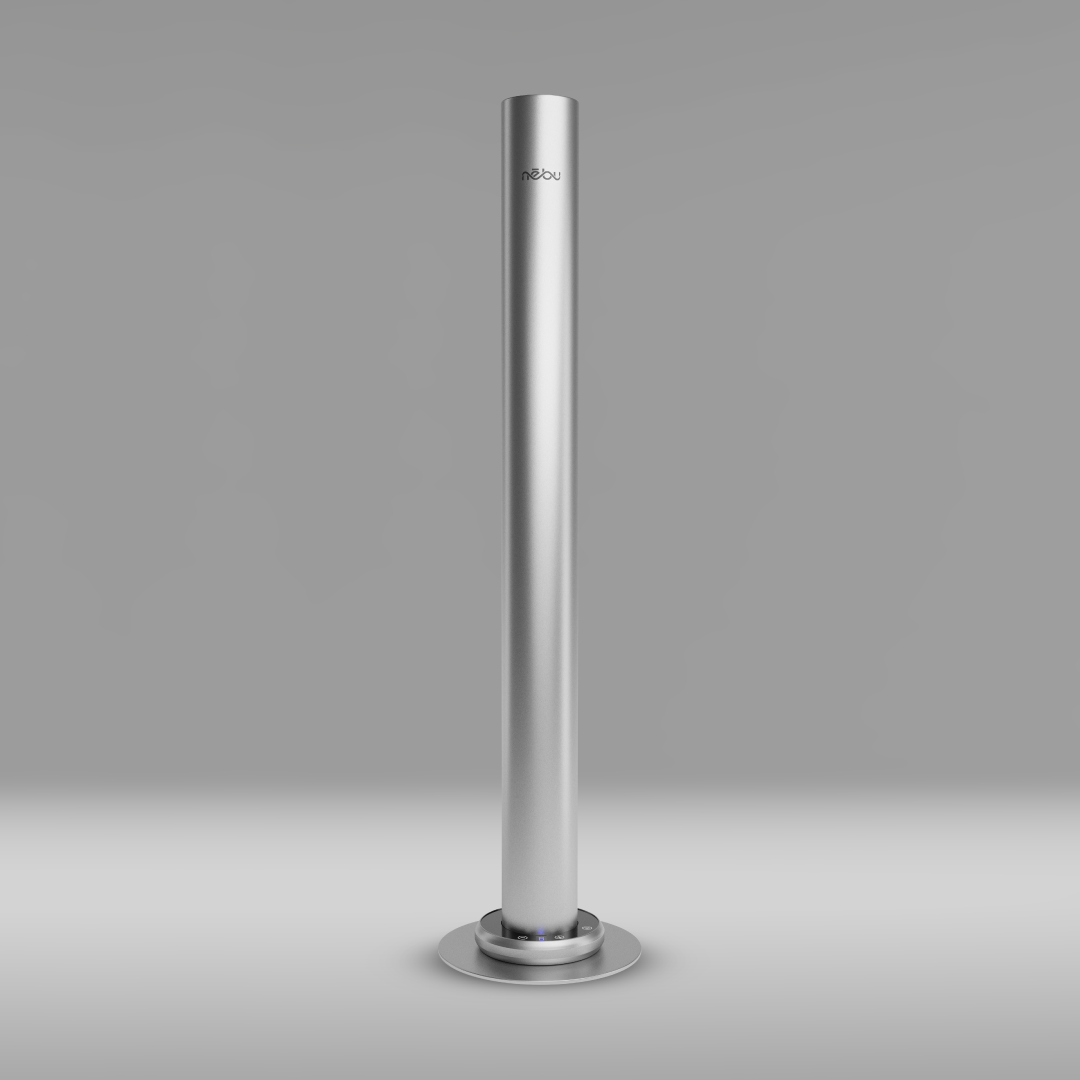The image depicts a tall, slender chrome cylinder standing prominently in the center. At the top of the cylinder, the word "Nebu" is inscribed in lowercase letters, with the letter "E" uniquely slanted to the left. The cylinder, roughly a foot in height, has a sleek and smooth surface, exuding a futuristic aesthetic. It is mounted on a base comprised of two circular rings: a smaller, thicker ring attached directly to the cylinder, which in turn sits on a larger, flatter ring. The background is predominantly monochromatic, with shades of gray transitioning from a darker hue at the top to a lighter one at the bottom, providing a subtle gradient that complements the metallic composition of the central object. There are no other texts or images present in the photo, highlighting the minimalistic and modern design of the scene.